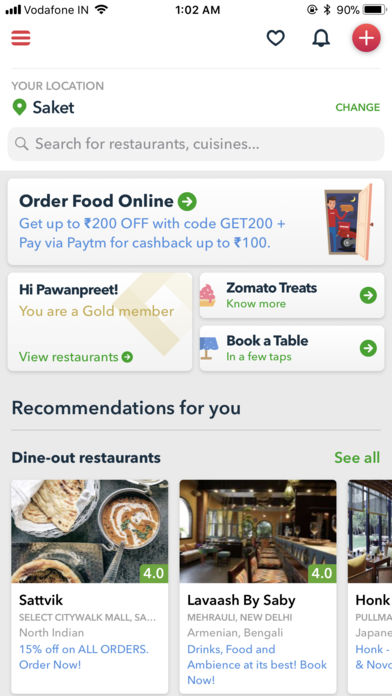**Screenshot from a Food Delivery App Interface**

The image depicts a screenshot taken on a phone displaying an interface from a food delivery app, likely captured in the early morning hours. The background is predominantly white.

- **Top Bar Information:**
  - Upper left corner displays cell phone coverage signal strength, Vodafone IN network indicator, and Wi-Fi signal strength.
  - In the center, the current time is shown as 1:02 AM.
  - Upper right corner shows various icons: battery percentage at 90%, Bluetooth symbol, and an indication that the phone screen orientation is locked.

- **Location and Search:**
  - Just below the top bar, there's a location text reading "Your location: Saket" with an option to change it by clicking a button to the right.
  - Directly beneath the location, there's a search bar inviting users to search for restaurants, cuisines, etc.

- **Promotional Banner:**
  - A promotional section advertises, "Order food online, get up to ₹200 off with code GET200 plus pay via PAYTM for cashback up to ₹100."

- **User Greeting and Options:**
  - To the right, a greeting message reads, "Hi Ponpreet," identifying the logged-in user as a gold member, followed by a link to view available restaurants.
  - The left section includes a few smaller tabs:
    - "Zomato Treats" 
    - "Know More" about Zomato Treats
    - "Book a Table" 
    - Additional options regarding the booking process.

- **Recommendations and Further Options:**
  - The lower section of the screenshot shows personalized recommendations under the heading "Recommendations for you."

The clean and organized layout ensures easy navigation, allowing users to seamlessly search, explore, and order from nearby restaurants.